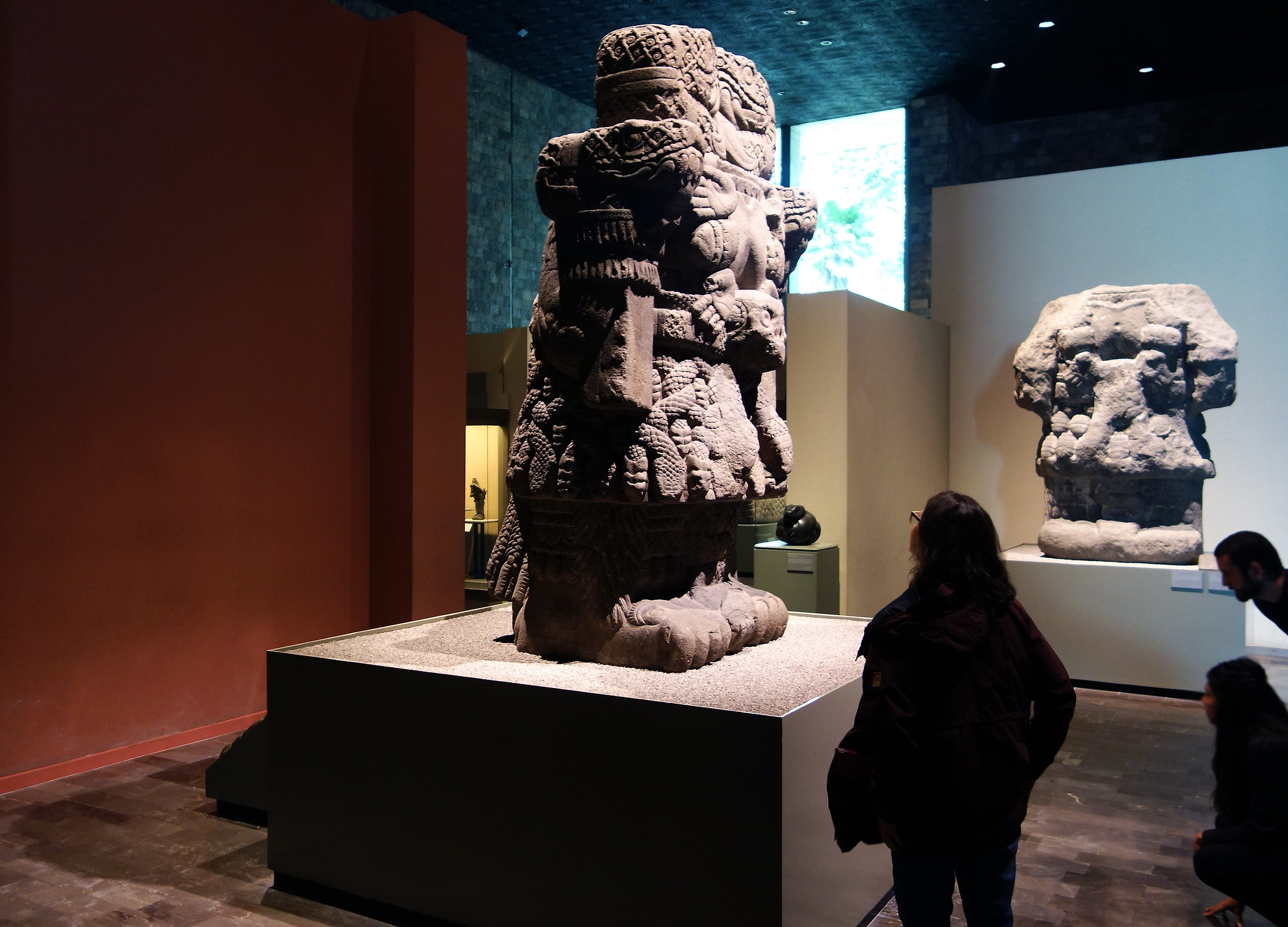In this photograph of a museum interior, we observe several ancient statues on display, likely transported from their original locations for preservation and exhibition. These statues depict humanoid figures with distinct anatomical exaggerations: prominent feet and skulls positioned centrally on their robust bodies. At the forefront of the image stands a relatively well-preserved statue, showcasing more intricate details than another, more eroded statue visible in the background.

Visitors to the museum are seen examining the exhibits, including a woman standing directly in front of the central statue. She is facing the display with her back to the camera, wearing glasses and a jacket, hands tucked into the jacket pockets, and her head tilted back as she gazes up at the statue's towering form.